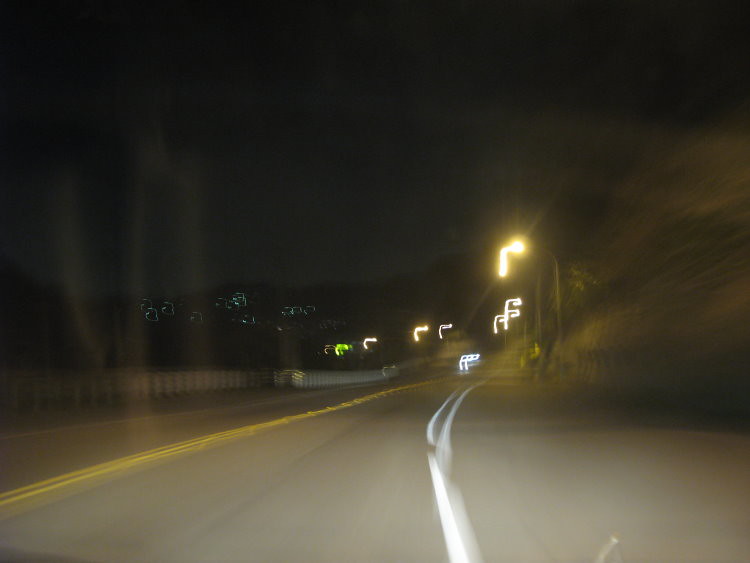The image captures a nighttime scene from within a moving vehicle, presumably in America, traveling down a two-lane road. The photograph, taken through the front windshield, shows a dark sky above. On the right side of the road, a blurry white line and grey road surface extend into the distance. A solid yellow line appears on the left, transitioning to a dotted line further ahead. On the left, a concrete wall or guardrail marks the road’s edge, accompanied by a visible fence. Blurry trees and a hill can be seen on the right side in the darkness. Overhead, arrow-shaped streetlights, casting a mix of yellow, white, and even a small green glow, are seen hanging from cables. These lights appear jagged due to the camera's motion. In the background, distant lights possibly from buildings suggest a residential or commercial area. An oncoming car approaches from the left lane, reflecting the glare from the windshield, adding to the blur.